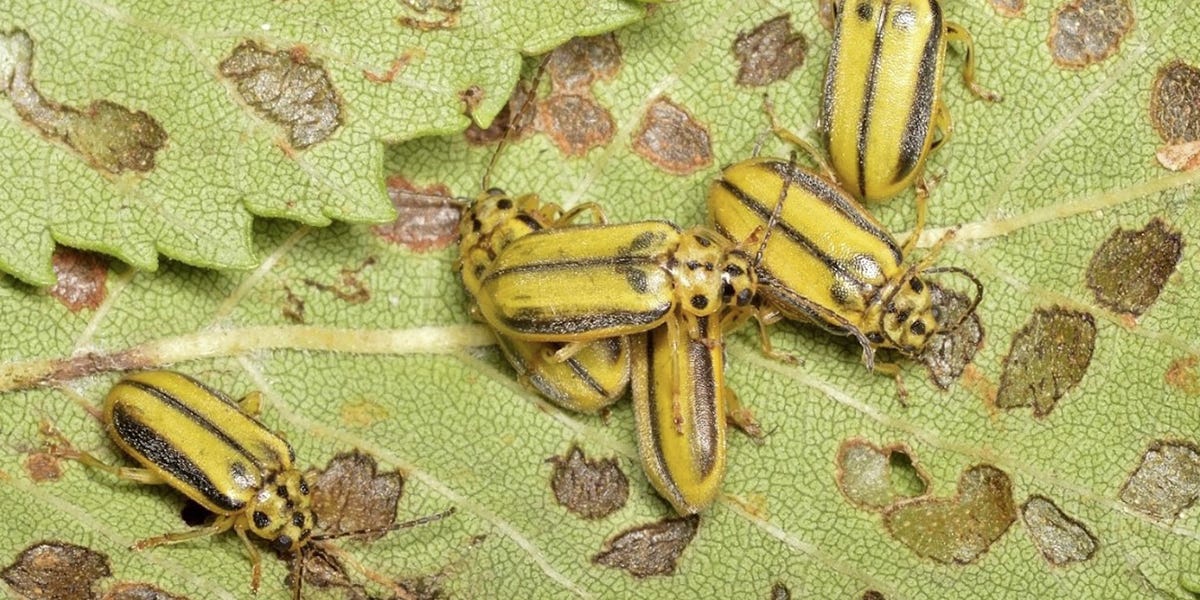The photo depicts several insects, likely beetles, resting on leaves. The leaves have a pistachio green hue and are marred with brown splotches. There are four to five oblong-shaped beetles, characterized by their yellow bodies with distinct black stripes running along the sides. Each beetle has antennae and six legs. The insects appear to have possibly caused some damage to the leaves, giving the impression they may have been feeding on them.